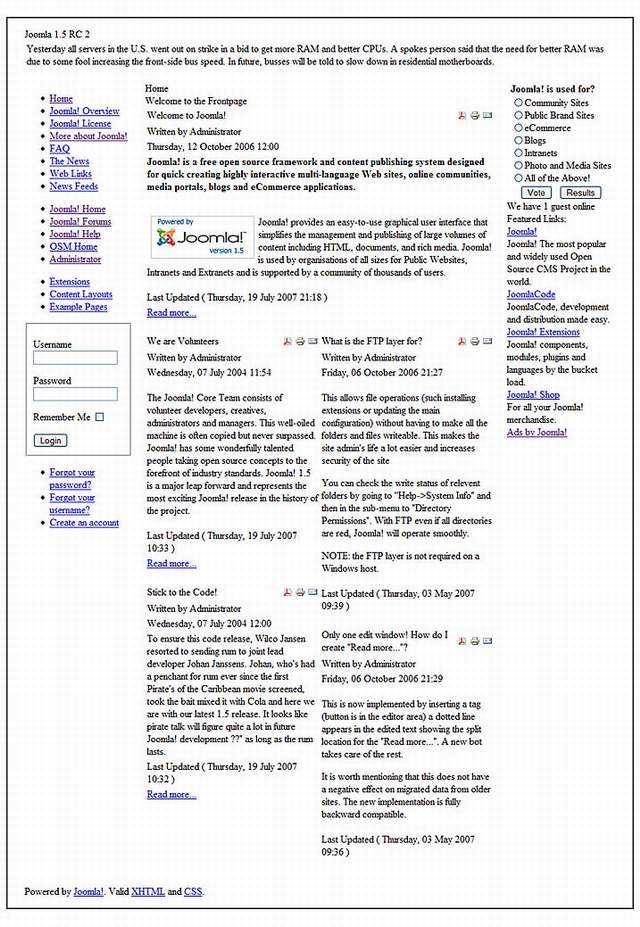Here is a detailed and cleaned-up descriptive caption:

---

The image features a white background with a central box that has a black border and a white interior. At the top of the box, black text reads: "Joomla 1.5 RC 2: Yesterday all servers in the US went out on strike in a bid to get more RAM and better CPUs. A spokesperson said that the need for better RAM was due to some full increase in the front side bus speed and future buses will be told to slow down on residential motherboards." 

Below this headline, it continues with the text: "Home. Welcome to the front page. Welcome to Joomla. Written by administrator on Thursday, 12 October 2006, 12:00 PM." 

Further down, the following description can be found: "Joomla is a free open-source framework and content publishing system designed for quickly creating highly interactive, multi-language websites, online communities, media portals, blogs, and e-commerce applications."

At the bottom of the box, there is another smaller white box centered with the text "Powered by Joomla" in the middle.

---